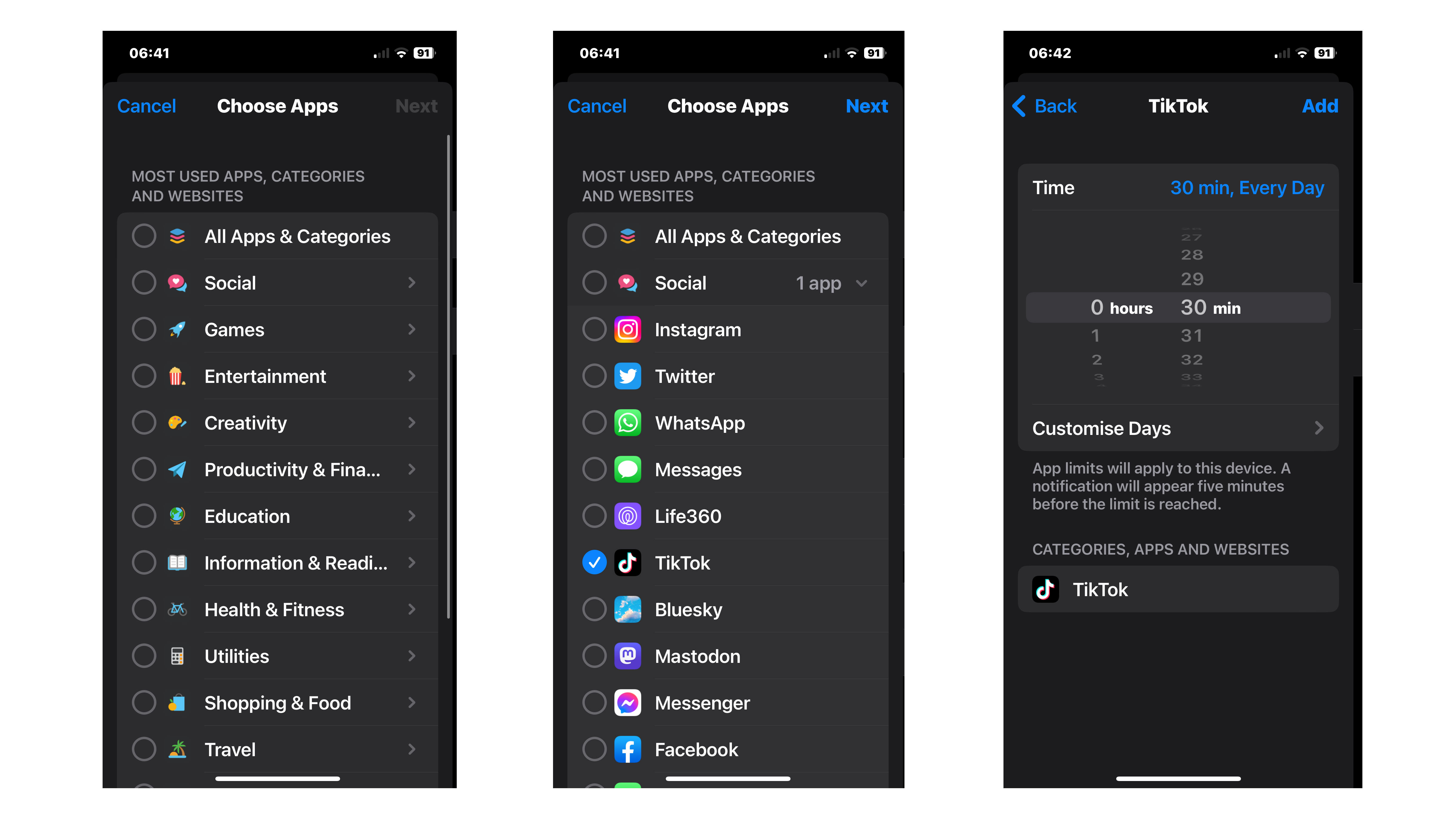Here is the cleaned-up and detailed caption for the image:

"The image showcases a smartphone interface, displaying various screens related to app usage management. At the top, '641' is prominently shown along with a battery indicator at 91%. A series of options for managing and categorizing app usage are visible, including buttons labeled 'Cancel' in blue, 'Choose Apps' in white, and 'Most Used Apps' in gray. The list includes categories like Social, Games, Entertainment, Creativity, Productivity and Fun, Education, Information and News, Health and Fitness, Utilities, Shopping, Food, and Travel. 

One of the screens features a detailed list of the social apps in use: Instagram, Twitter, WhatsApp, Messages, Live Thread 60, TikTok, Mastodon, Messenger, and Facebook. It also includes a timer setting allowing users to limit app usage to 30 minutes every day, with customized dates and notifications appearing 5 minutes before the limit is reached. The current time shown is 6:42 PM. Overall, these screens highlight the smartphone’s comprehensive app management and usage tracking features."